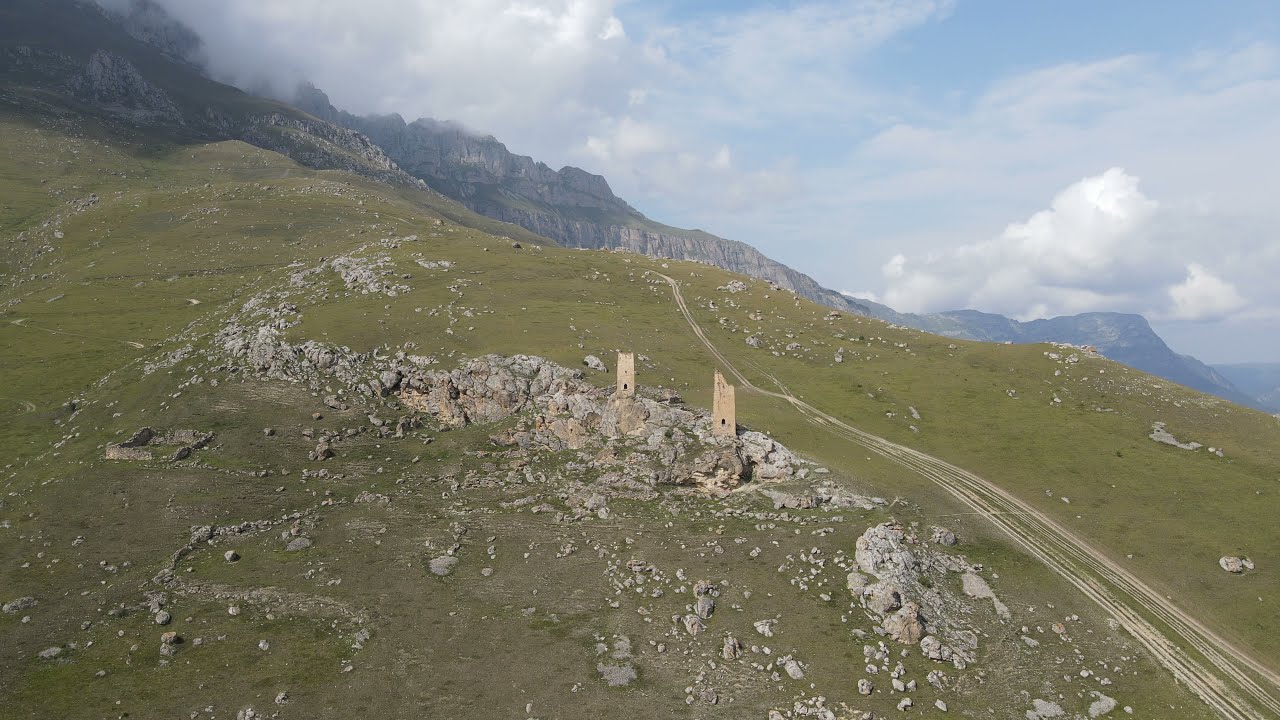The photograph depicts a scenic, mountainous landscape taken during a partly cloudy day. Dominating the left side of the image, there are the ruins of what appears to be an old castle or fortification, including two crumbling, tan stone towers with dark window openings, standing amidst a field of short, dark green grass interspersed with white rocks. These ruins are situated on a rocky outcrop. A dirt path or road begins at the lower right corner and meanders through the scene, leading towards the center background, giving a sense of depth and guiding the viewer's eye through the landscape. The terrain becomes increasingly rocky and elevated towards the top of the image, where jagged mountain peaks rise and blend into a sky filled with white clouds and patches of blue. The highest peaks are partially obscured by these clouds, emphasizing the altitude and grandeur of the scene. The sunlight filtering through the clouds adds a touch of brightness to the predominantly green and gray palette of the mountainside.